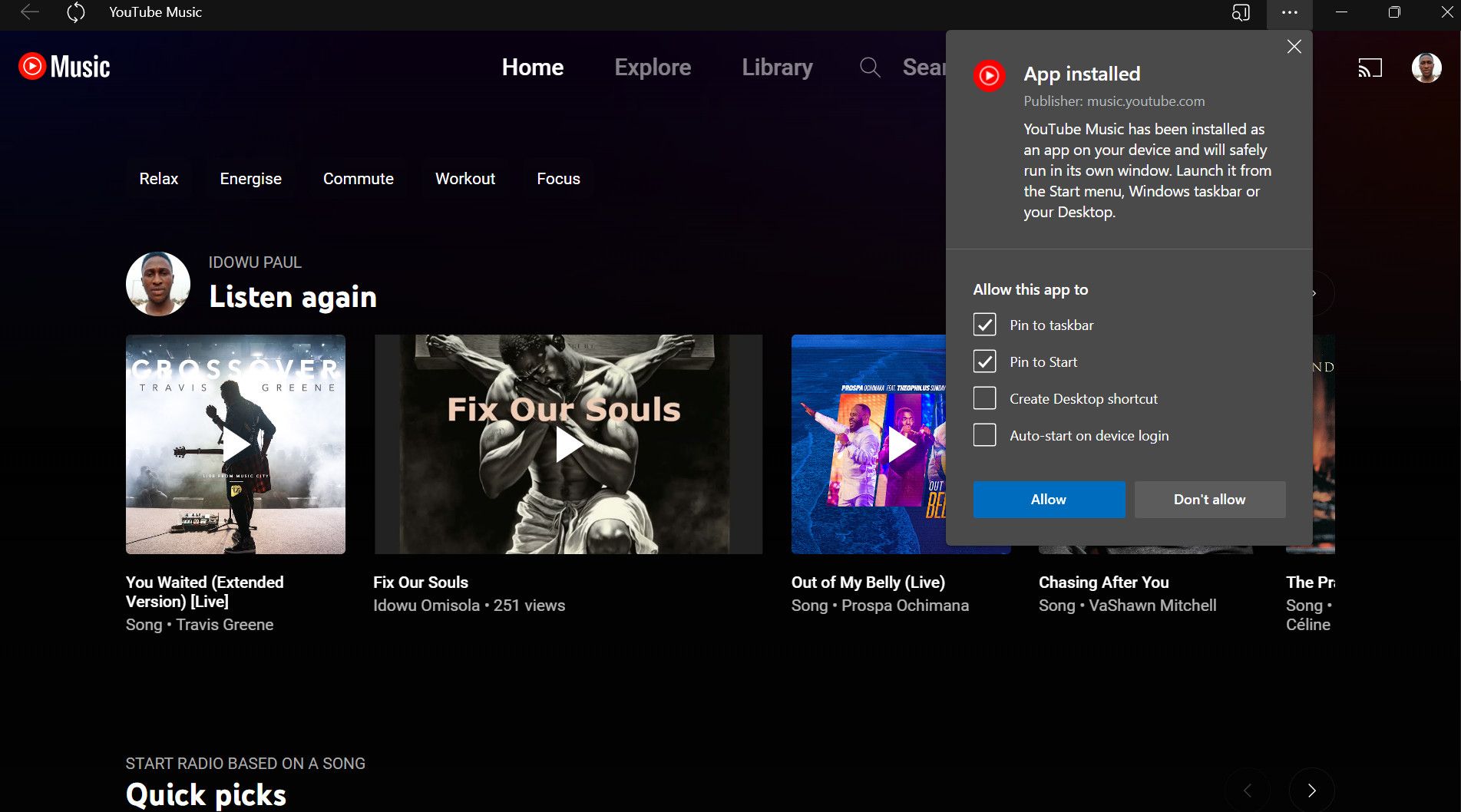In the image, we see a detailed snapshot of the YouTube Music app, closely resembling a YouTube Music Premium interface. At the upper left corner is the "YouTube Music" text in white. Adjacent to it, a reload button and the iconic YouTube Music logo—featuring a red circle encasing a white triangle pointed to the right, representing a play button, with a capital 'M' for Music.

The interface menu spans across the top with options: Home, Explore, Library, and Search. Below, a pop-up notification indicates "YouTube Music app installed" with the publisher listed as music.youtube.com. This notification elaborates that YouTube Music has been installed on the device and will run in its own window. It offers options for the user: pin to taskbar, pin to start, create a desktop shortcut, and auto-start upon the next device login.

Towards the left side, there is a category menu featuring different music types: "Relax," "Energize," "Commute," and "Workout and Focus". A user profile for "Idau Paul" is displayed, with a "Listen Again" section showcasing four boxes of different artists for easy access and replay.